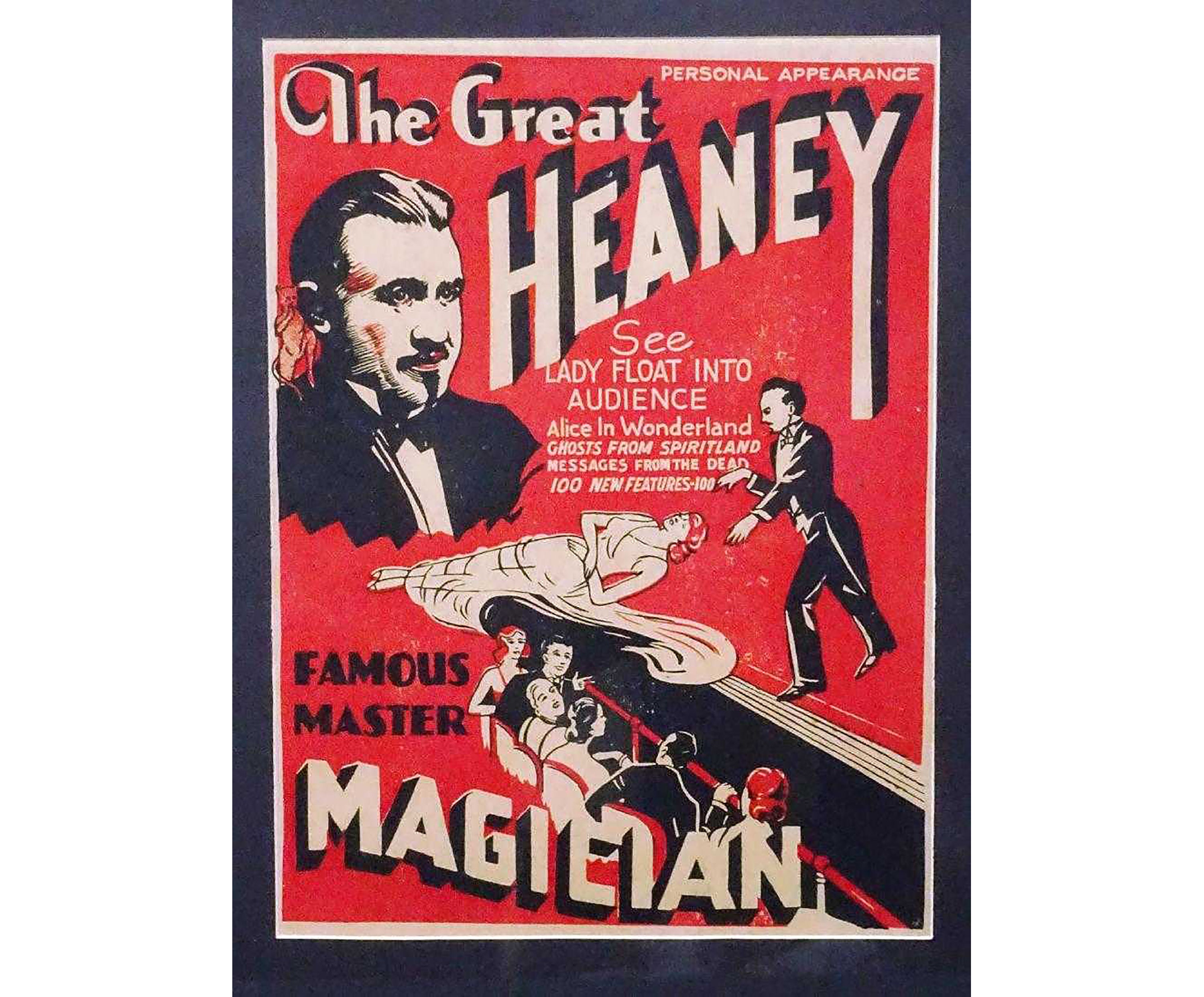This vibrant, hand-drawn vintage poster, likely from the early 1900s, advertises a spellbinding magic show by "The Great Heaney." Set against a striking red background, the text at the top is rendered in bold, 3D-like letters, spelling out "The Great Heaney." To the top right, "Personal Appearance" is prominently displayed. The poster is detailed with multiple phrases promising astounding feats: "See Lady Float into Audience," "Alice in Wonderland," "Ghosts from Spirit Land," "Messages from the Dead," and "100 New Features."

In the top left corner of the poster, there is a detailed illustration of The Great Heaney himself. He has slicked-back black hair, a mustache, and a goatee that stripes down the middle of his chin. He is also impeccably dressed in a tuxedo with a black jacket, white collared shirt, and a black bow tie. Interestingly, a small mouse appears to be whispering into his ear from his shoulder.

The middle of the poster features another captivating scene: Heaney, dressed in his signature tuxedo, performs a levitation act with a woman in a dress lying horizontally above the ground. An audience is depicted in the background, seated and seemingly mesmerized by the spectacle.

At the bottom of the poster, the text proclaims Heaney as the "Famous Master Magician," cementing his legendary status in the world of magic.